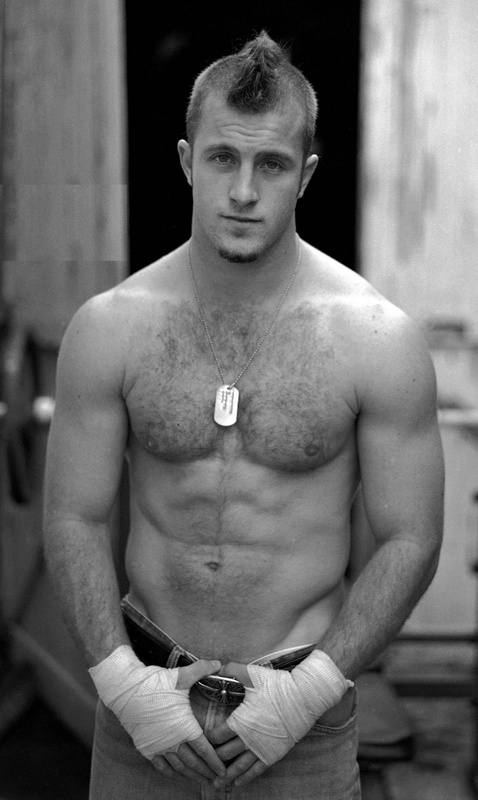The grayscale image features a shirtless male, identified as Scott Kahn, posing confidently at the camera. He sports a defined physique, highlighted by his pronounced abs and muscular forearms, which are slightly hairy. His distinct style includes a mohawk and a very thin goatee on his chin, with no other facial hair. Around his neck, he wears a military dog tag.

The man’s thumbs are tucked into his belt loops, slightly pulling down his jeans, which are fastened with a belt. His hands are taped with white tape, suggesting a readiness for a fight, reminiscent of a UFC fighter. The indoor setting is blurry, with some indistinguishable objects possibly including exercise equipment in the background. The floor appears to be carpeted, although it is also somewhat unclear. There is a doorway and walls visible in the background, which further emphasize the indoor environment. The absence of color in the image leaves everything rendered in shades of black, white, and gray. The overall impression is that this shoot could be for a fitness or underwear magazine, exuding a rough and tough persona.